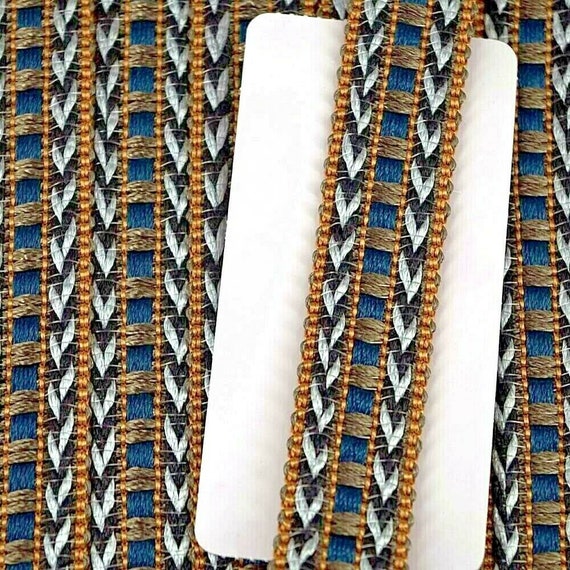This highly detailed, square photograph captures a vertically aligned, ornately braided ribbon that appears to be wrapped around a flat surface for display. The ribbon features a complex pattern with a center strip sporting blue stitching interwoven with medium brown to create a checkerboard effect, and flanked by thin gold lines. On either side of this central section are strips of black and white herringbone stitching, with the arrows of the herringbone pattern pointing downward and lined with gold beads. The image also shows a rectangular white business card-shaped piece of paper with rounded corners tucked behind the foremost strip of the ribbon, highlighting the intricate borders and adding contrast to the overall display. Approximately six to seven strands of this pattern are visible, showcasing the repetitive and meticulous design of the ribbon.